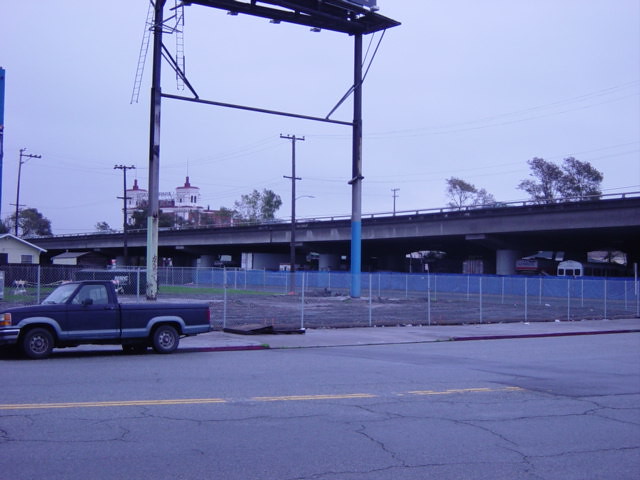In this daylight photograph, an outdoor scene is captured with a distinct bluish tint. The sky is impeccably clear, painting a tranquil blue backdrop. In the foreground, an aged street can be seen, characterized by cracks and an eroded yellow line running down its center. An old pickup truck, possibly from the 1980s, is parked at the curb, showcasing dark blue paint with silver trim. 

Further in the background, silver and blue gates are visible, leading to an elevated freeway. Adjacent to the freeway, the structure of a billboard is discernible, its metal supports rising up to the platform, although the advertisement remains unreadable. 

The horizon is lined with several power lines, numbering at least five or six. A white brick building with distinctive turrets stands prominently beyond, adding architectural interest. Additionally, a house is also present within the frame, contributing to the detailed urban landscape.